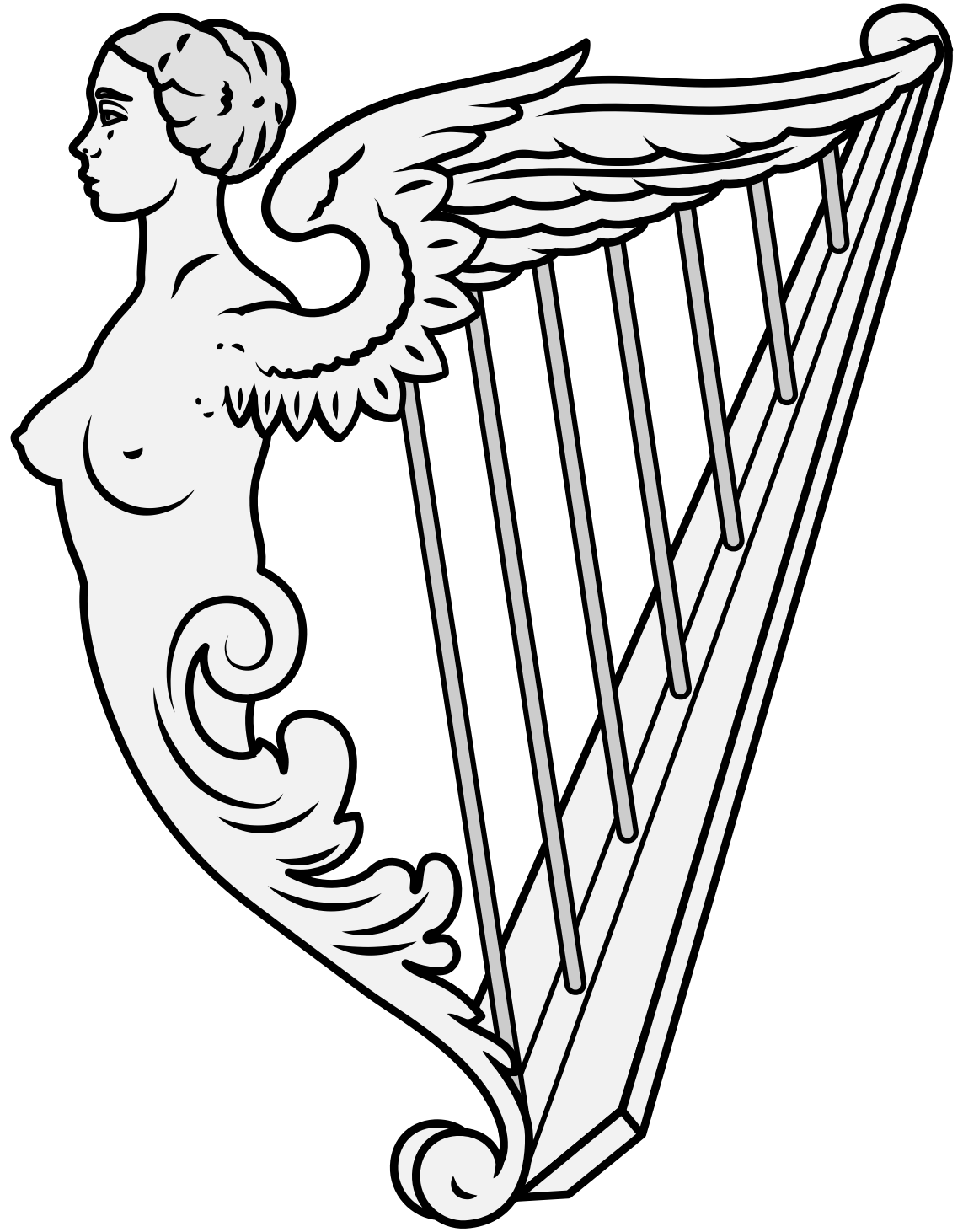A black-and-white hand-drawn illustration depicts an intricately detailed harp with a clip art style. The majority of the harp's structure integrates the bust of a bare-chested female angel, whose short hair is styled in a bun. Her serene expression contrasts with the ornate complexity of her form, which transitions from her torso into the harp's composition. The top part of the harp is shaped by one of the angel's bird-like wings, while her lower body morphs into an elaborate design resembling a seahorse fin, forming the side of the instrument. The harp features a standard base connecting the tail and the wing, and there are seven thick strings or chords spanning from the angel's back to the opposite end, which appear more like ropes than traditional harp strings.